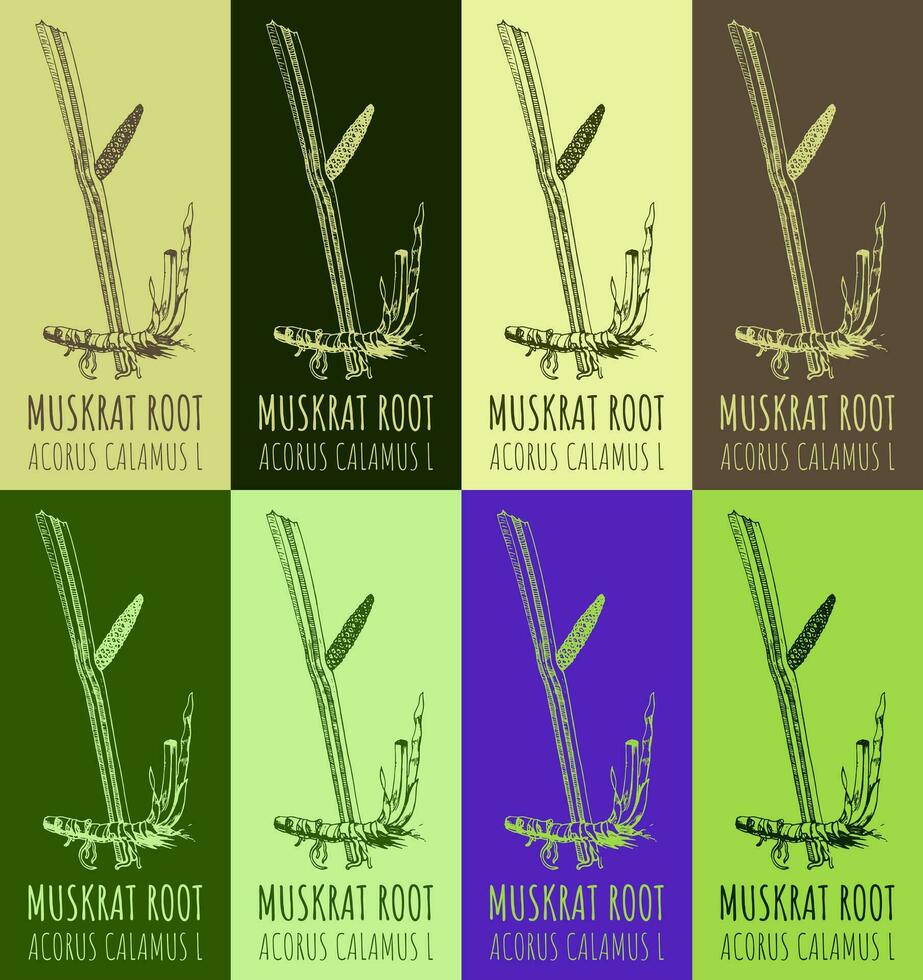The image is an advertisement or pop art poster featuring eight individually squared graphics, arranged in two rows with four graphics at the top and four at the bottom. Each graphic displays the same illustration of a plant called muskrat root, labeled with the text "muskrat root" and the scientific name "Acorus calamus L." The plant image consists of a stocky shoot emerging from a central, curved root, with a smaller shoot pointing upward.

Each graphic has a unique background color, distinguishing them from one another. The top row features backgrounds in light green, dark brown, creamy green, and medium brown. The bottom row has backgrounds in dark green, lime green, dark blue, and bright light green. This repeated motif with varying background colors forms a visually intriguing and cohesive poster design.